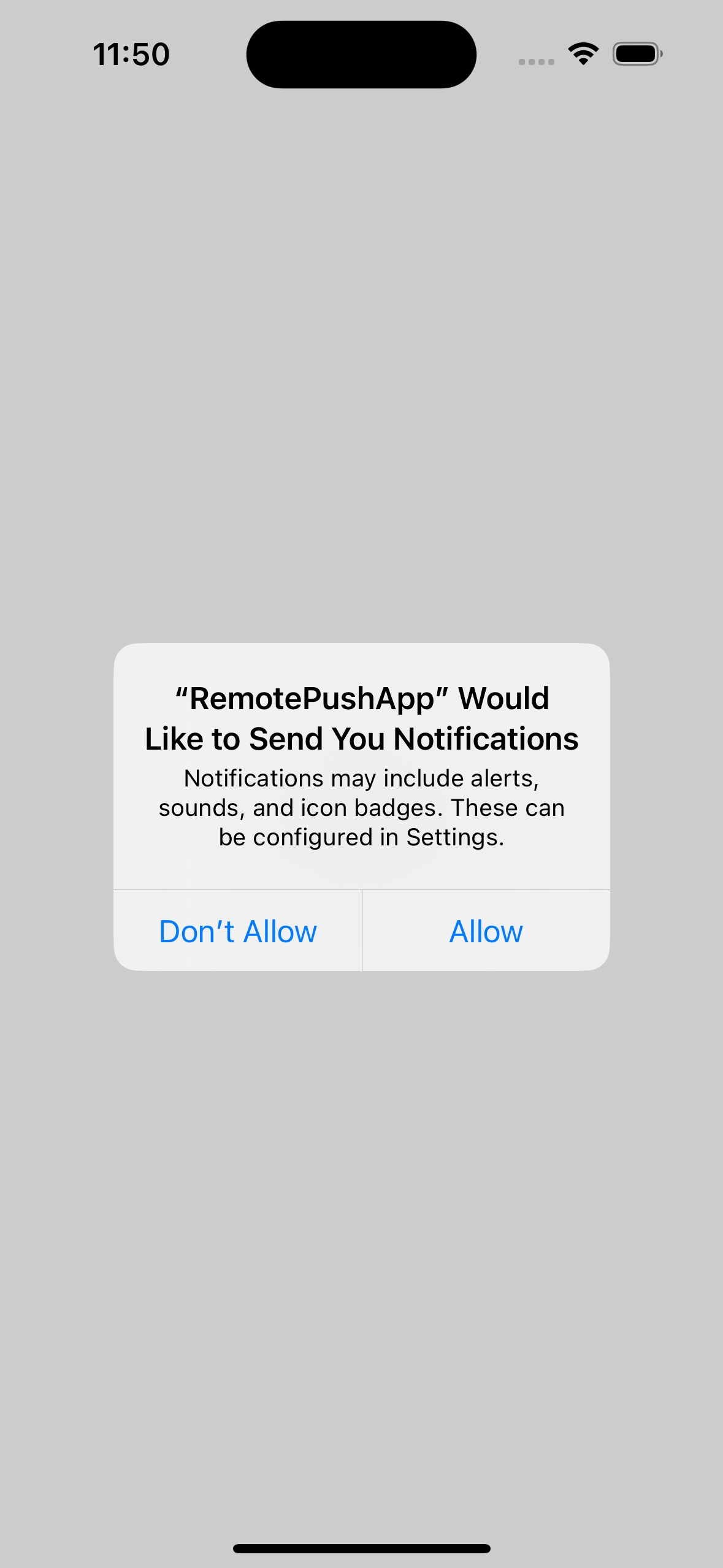The image depicts a cell phone screenshot with a background of solid medium gray. The screenshot's aspect ratio is approximately three times as high as it is wide. 

In the upper left corner, the current time is displayed as 11:50 in black text. At the top center of the screen, there is a black, centrally-located oval-shaped icon with rounded sides. To the right of this icon, there are four gray dots and a signal strength indicator showing three out of three bars. The battery icon, also located at the top, indicates a full charge.

Prominently centered in the middle of the image, both vertically and horizontally, is a gray rectangle with rounded edges. Inside the rectangle, in large, bolded black text, is the message: 

"RemotePushApp" (each word within this compound word starts with a capital letter). Below this in smaller, bold text, the notification reads, "Would Like to Send You Notifications" (with each word capitalized).

Further down in even smaller text, the message elaborates, "Notifications may include alerts, sounds, and icon badges. These can be configured in settings."

At the bottom of the gray rectangle are two options in smaller text: "Don't Allow" in light blue on the lower left side, and "Allow" in light blue on the lower right side.